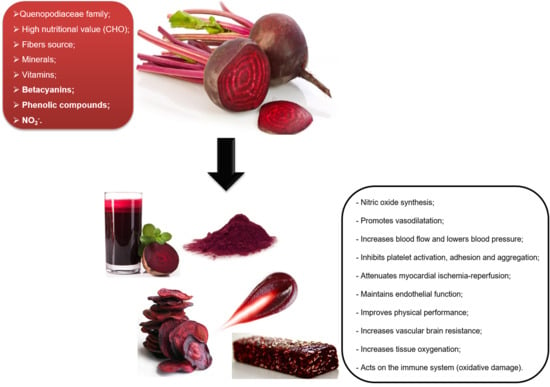This full-color infographic, set against a minimalist white background, illustrates the various properties and uses of beets. In the upper section, two beets are shown: one is uncut with a green leaf, and the other is sliced vertically to reveal red interior slices. A downward-pointing black arrow connects these beets to an array of beet-derived products below. Directly beneath the arrow is a pile of beet fragments, indicative of beet processing. To the left of the fragments, there's a cup filled with red beet juice, and to its right, a red bar, suggesting a beet-based snack. The infographic includes detailed annotations: in the upper left, inside a red square, it highlights the nutritional benefits—fiber source, minerals, vitamins, and various compounds such as beta-cyanines and phenolic compounds, emphasizing the high nutritional value of beets. Along the lower right, more detailed text specifies health benefits including nitric oxide synthesis, improved vasodilation, increased blood flow, lowered blood pressure, reduced platelet aggregation, enhanced physical performance, increased tissue oxygenation, and boosted immune function.